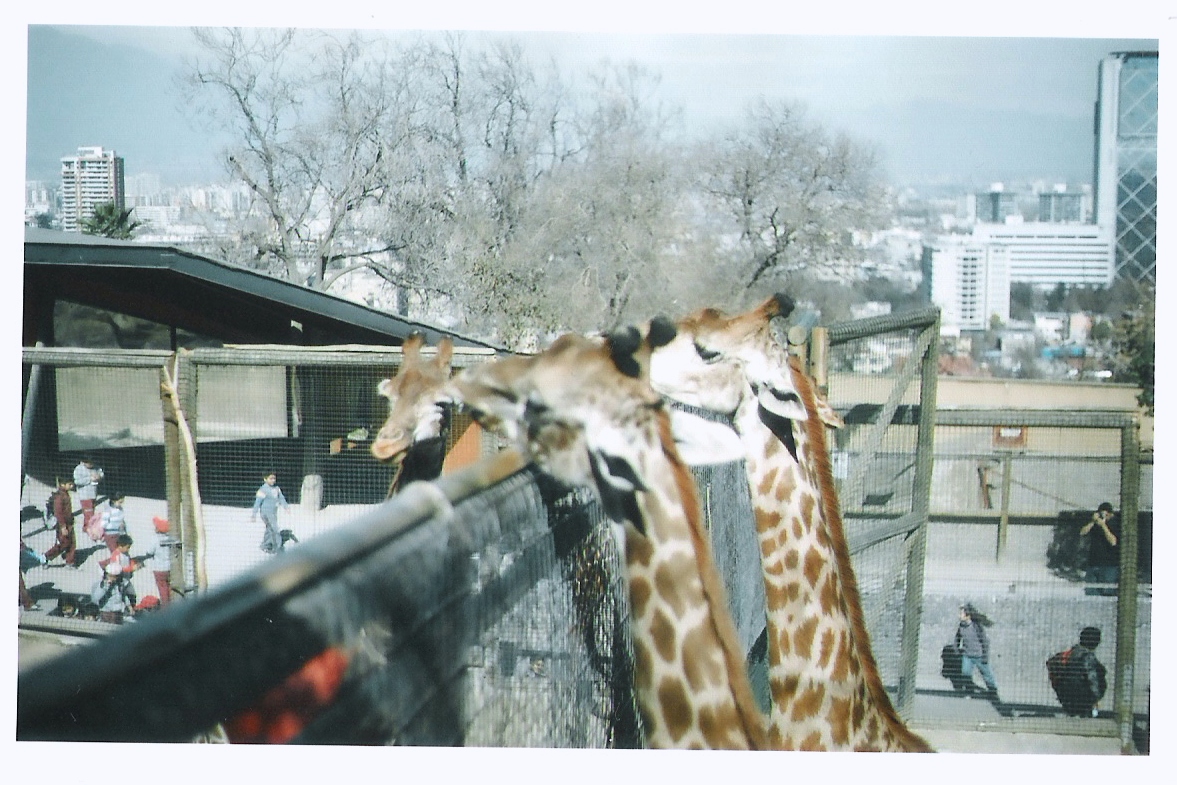An outdoor color photograph taken in bright daylight captures a zoo setting with a focus on a group of giraffes. Central to the image are their long necks and heads, with two giraffes prominently shown in profile in the center. Another giraffe is slightly to the left, tilting its head to the right. All giraffes are positioned next to a tall chain-link fence, with only their necks and heads visible. The giraffes exhibit ivory bodies with medium tan splotches and varying shades of brown on their noses and ears. 

In the foreground, children and a few adults are visible, including a parent taking photographs. The fence extends from the lower left corner toward the center, with another fence further in the background. Beyond the enclosure, a sprawling, slightly hazy cityscape marked by high-rise buildings is visible. The background also includes bare, leafless trees indicative of winter. Among the structures, a black building with a gray roof and a few other buildings add to the urban setting. 

Overall, the photograph provides a detailed and layered view of the zoo environment, blending the natural appeal of the giraffes with the bustling human activity and the encompassing urban landscape.